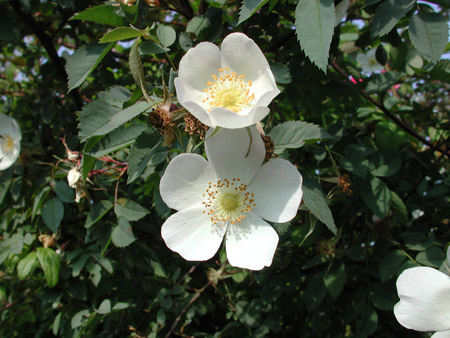In this vibrant outdoor photograph, the focal point is a cluster of striking white flowers growing amidst a lush green bush. The largest and most opened flower sits prominently in the center, showcasing its five broad white petals that taper towards a yellow-green center, from which orange-tipped stamens emerge. Directly above it, another flower of the same kind is partially open, hinting at its pending full bloom. The scene also includes two more identical flowers, one peeking from the top left corner and another from the bottom right, hinting at the abundance of blooms within the bush. Surrounding the flowers are dark green leaves with jagged, tooth-like edges, creating a rich, textured backdrop. Between the foliage, glimpses of blue sky and hints of red plants add depth and color contrast to the composition.